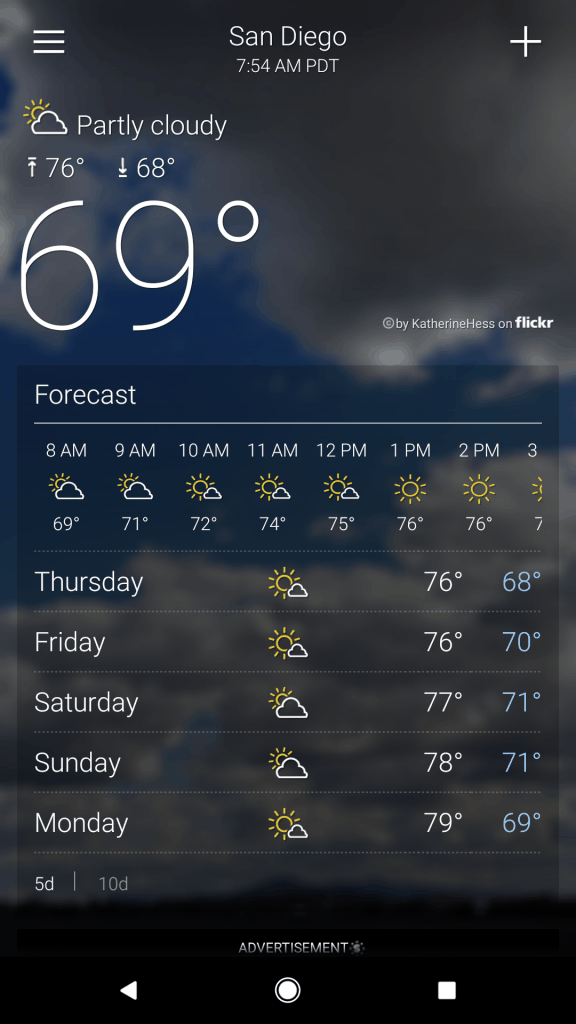Screenshot of a weather app on a phone, displaying the forecast for San Diego, taken at 7:54 a.m. PDT. At the top of the screen, "San Diego" is prominently displayed, indicating the location. To the left, there's a menu icon represented by three horizontal lines, while a cross icon on the right suggests options to close or exit. Below the location, it states "Partly Cloudy" accompanied by an icon showing a white cloud and a yellow sun.

The current temperature is prominently displayed as 69°F, with an expected high of 76°F and a low of 68°F for the day. The detailed forecast chart lists hourly temperatures starting from 8 a.m. through 3 p.m., though the 3 p.m. forecast is partially cut off. Most of the hourly updates indicate sunny conditions, with occasional clouds.

A further detailed five-day forecast lists:
- **Thursday:** High of 76°F, low of 68°F
- **Friday:** High of 76°F, low of 70°F
- **Saturday:** High of 77°F, low of 71°F
- **Sunday:** High of 78°F, low of 71°F
- **Monday:** High of 79°F, low of 69°F

At the bottom of the screen, there are options for viewing five-day and ten-day forecasts, followed by the word "Advertisement," indicating the presence of ads on the app.

The image caption credits Catherine Hess on Flickr as the source.